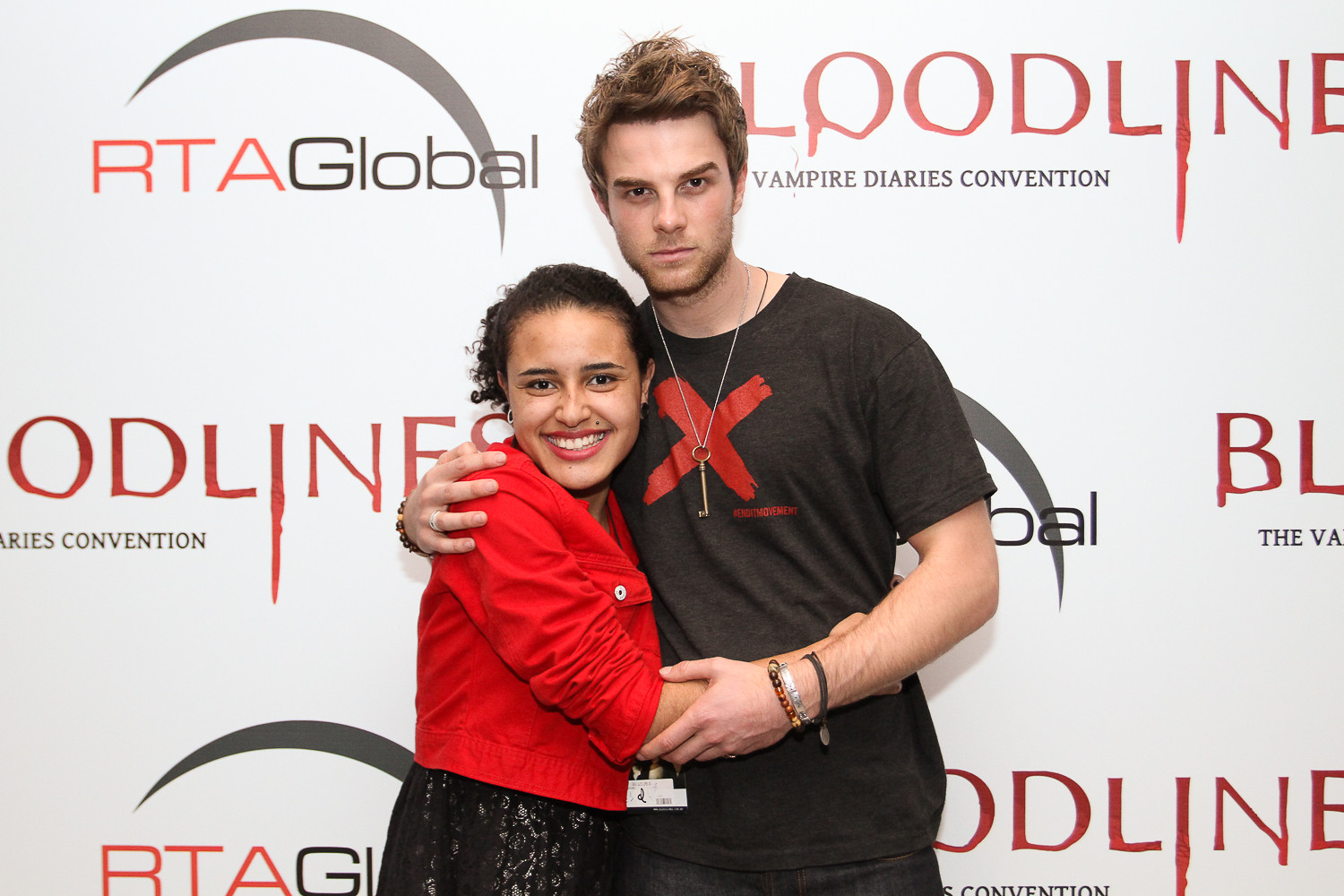In the photo, a young man and woman are standing in front of a large, white billboard with a blood-dripping "Bloodline" logo and accompanying text, indicating it's for the Vampire Diaries Convention, mentioning a sponsorship by RTA Global which is repeated throughout the backdrop. The woman, who appears to be of Indian descent, has her dark hair up in a ponytail and wears a black skirt paired with a red long-sleeve shirt or possibly a short jacket with sleeves pushed up. She smiles brightly at the camera. The man beside her, likely in his mid-twenties, has blondie-brown hair with dark roots, a short beard, and wears dark pants with a black short-sleeve t-shirt bearing a red X across the chest. He's accessorized with several bracelets on his left arm and a chain necklace holding a large, old-fashioned key. He gazes seriously into the camera while his right arm is wrapped around the woman in a half-hug pose.